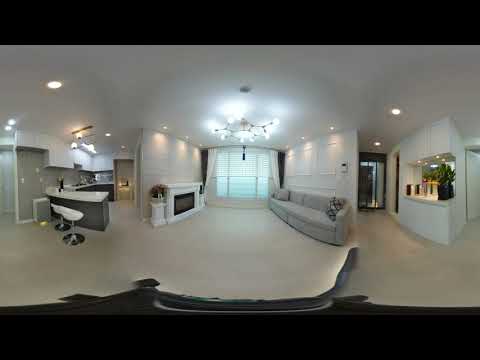This detailed panoramic photograph captures the airy and modern interior of a light-colored home, seamlessly blending three distinct spaces. On the left side, there is a sleek, contemporary kitchen featuring dark gray cabinets and white countertops. It boasts an island bar setup with two white stools, modern pendant lights hanging above, and additional countertop space adorned with plants. The center of the image reveals a minimalist living room, characterized by a gray couch positioned against the right wall and a sophisticated white mantel and fireplace on the left. Above, a striking chandelier resembling branches with light bulbs adds a touch of artistic flair. To the right, there is a small hallway with a cut-out window ledge displaying decorative items, leading to a doorway to another room and a closet door. The walls throughout are pristinely white, and the ceiling is dotted with spotlights, enhancing the spacious and well-lit ambiance of the home.